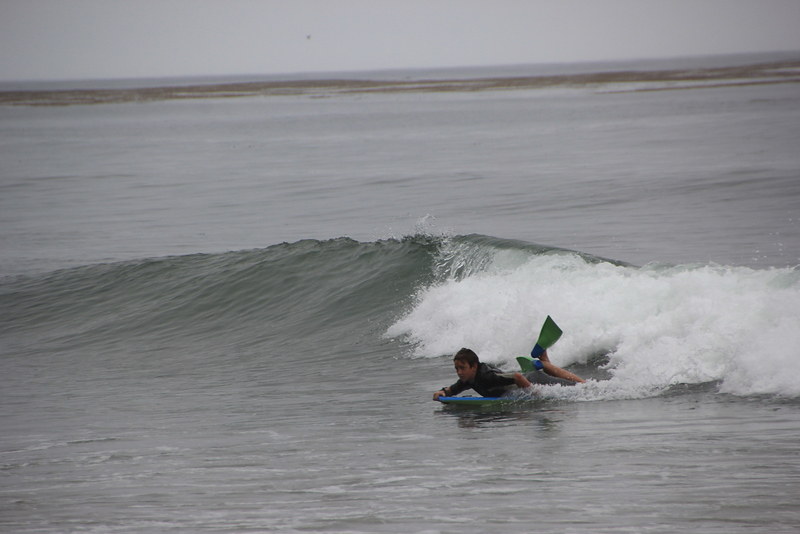This detailed photograph captures a person, ostensibly male with caramel-colored skin and dark hair, engaged in boogie boarding amidst rolling ocean waves. The focal point of the image is the individual, centered but slightly lower in the frame, lying on a vibrant blue boogie board as they ride a crashing wave. They are equipped with a sleek black wetsuit and distinctive flippers that are green towards the toes and blue towards the heels, harmonizing with the boogie board. The wave they are riding is foaming and crashing to the top right of the person, adding dynamic energy to the scene. The ocean water surrounding them exhibits a muted bluish-green hue, while the breaking waves introduce splashes of white foam. In the backdrop, the horizon displays a stretch of indistinct brown land beneath an overcast gray sky, which occupies the upper eighth of the image. The combined elements convey a vivid yet serene moment of enjoyment and adventure in the ocean.